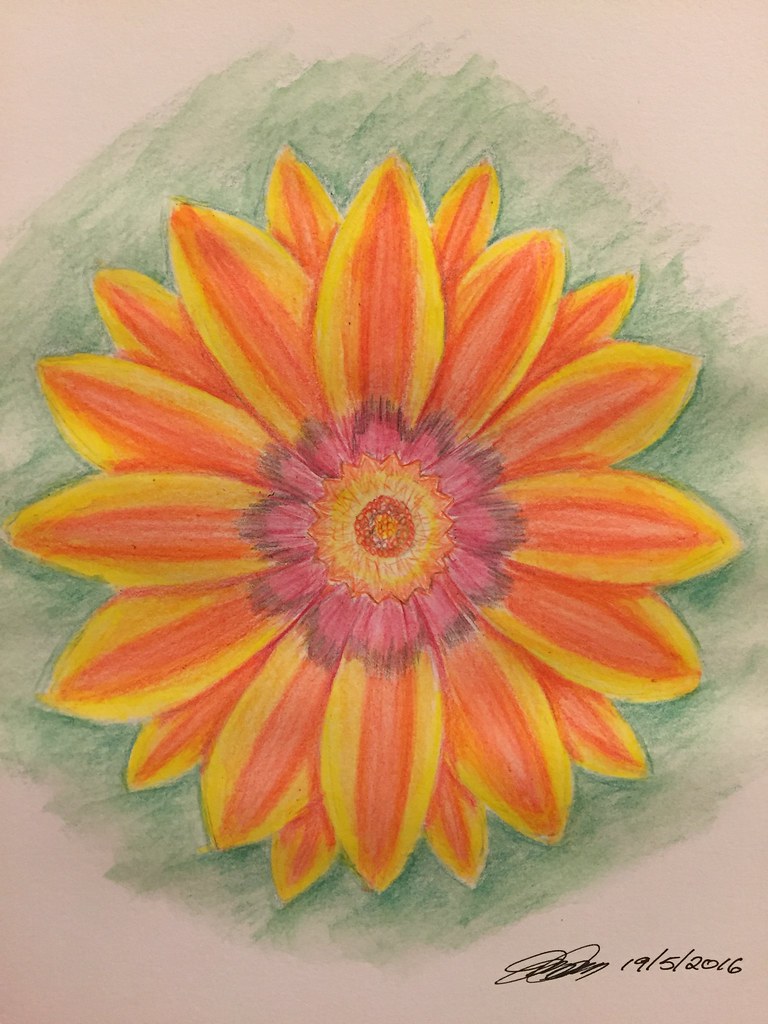This is a highly detailed pencil drawing of a flower, set against a delicate pale tannish-peach background. Dominating the center of the composition is the flower itself. At the heart of the flower lies a small circle comprised of minuscule dots in shades of orange, yellow, and a hint of white. Surrounding this central circle is an outer ring, which features a gradient of yellow, orange, and white that intensifies in color toward the edge. 

Beyond this ring, we encounter the beginning of the petals, which are characterized by a pale red hue accentuated by fine, light black lines extending from the outer edges. The petals, reminiscent of those found on a daisy, are primarily yellow with a peach core outlined in orange. Soft green shading envelops the entire flower, adding depth and a touch of realism.

In the bottom right corner of the drawing, the artist's black signature and date are discretely inscribed, completing the artwork with a personal touch.